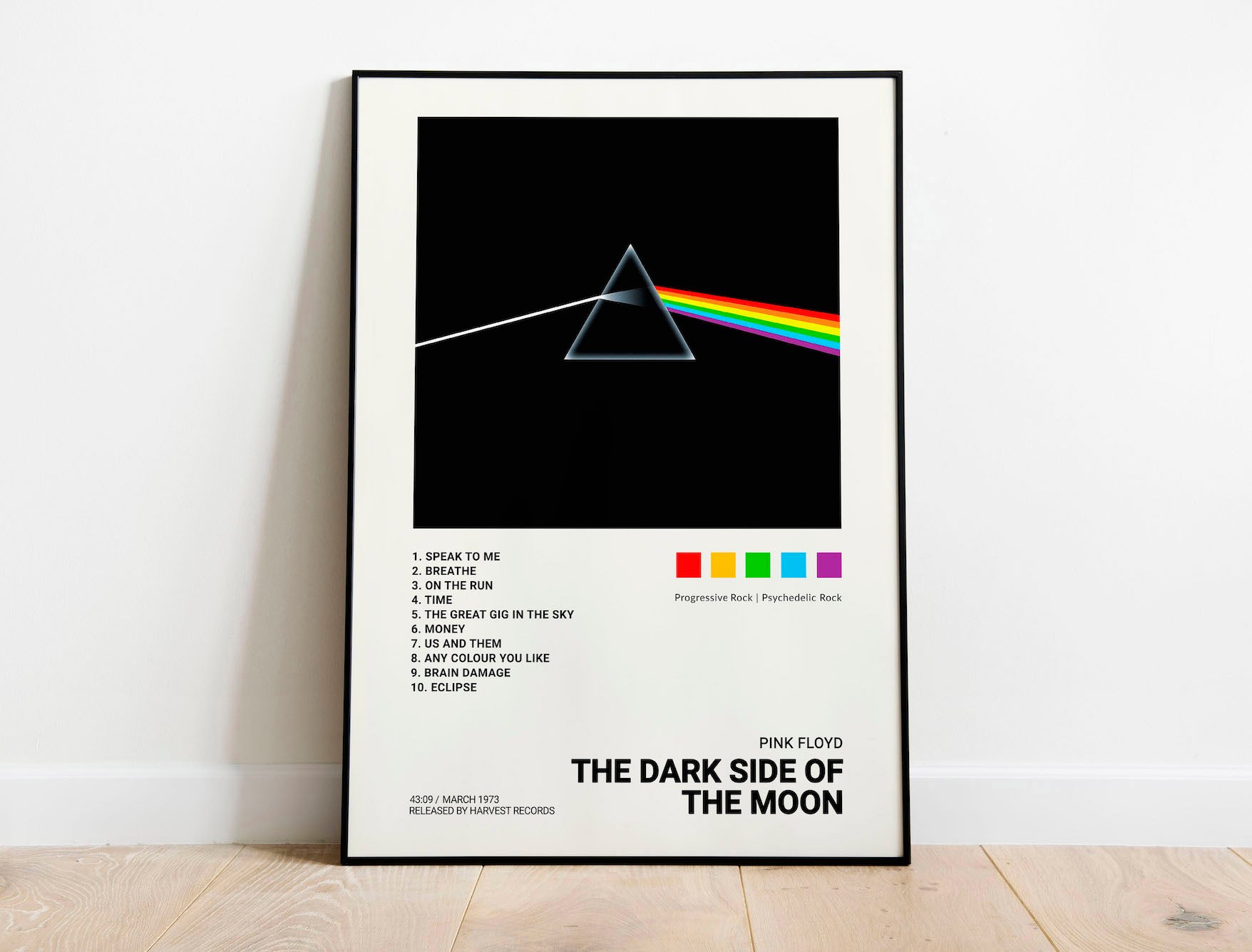This photograph features a framed poster leaning against a wall. The poster is an advertisement for Pink Floyd's iconic 1973 album, The Dark Side of the Moon. The image replicates the album's cover art, showcasing a black background with a white-outlined triangle. A stream of white light enters the prism from the left, transforming into a vibrant rainbow as it exits on the right, displaying the colors red, yellow, green, blue, and purple. Below the prism, the poster lists the ten tracks from the album: 1. Speak to Me, 2. Breathe, 3. On the Run, 4. Time, 5. The Great Gig in the Sky, 6. Money, 7. Us and Them, 8. Any Colour You Like, 9. Brain Damage, and 10. Eclipse. The text mentions the genres "progressive rock" and "psychedelic rock," with little color swatches underlining these descriptors. The release date, March 1973, is also highlighted, adding to the poster's historical and cultural significance.